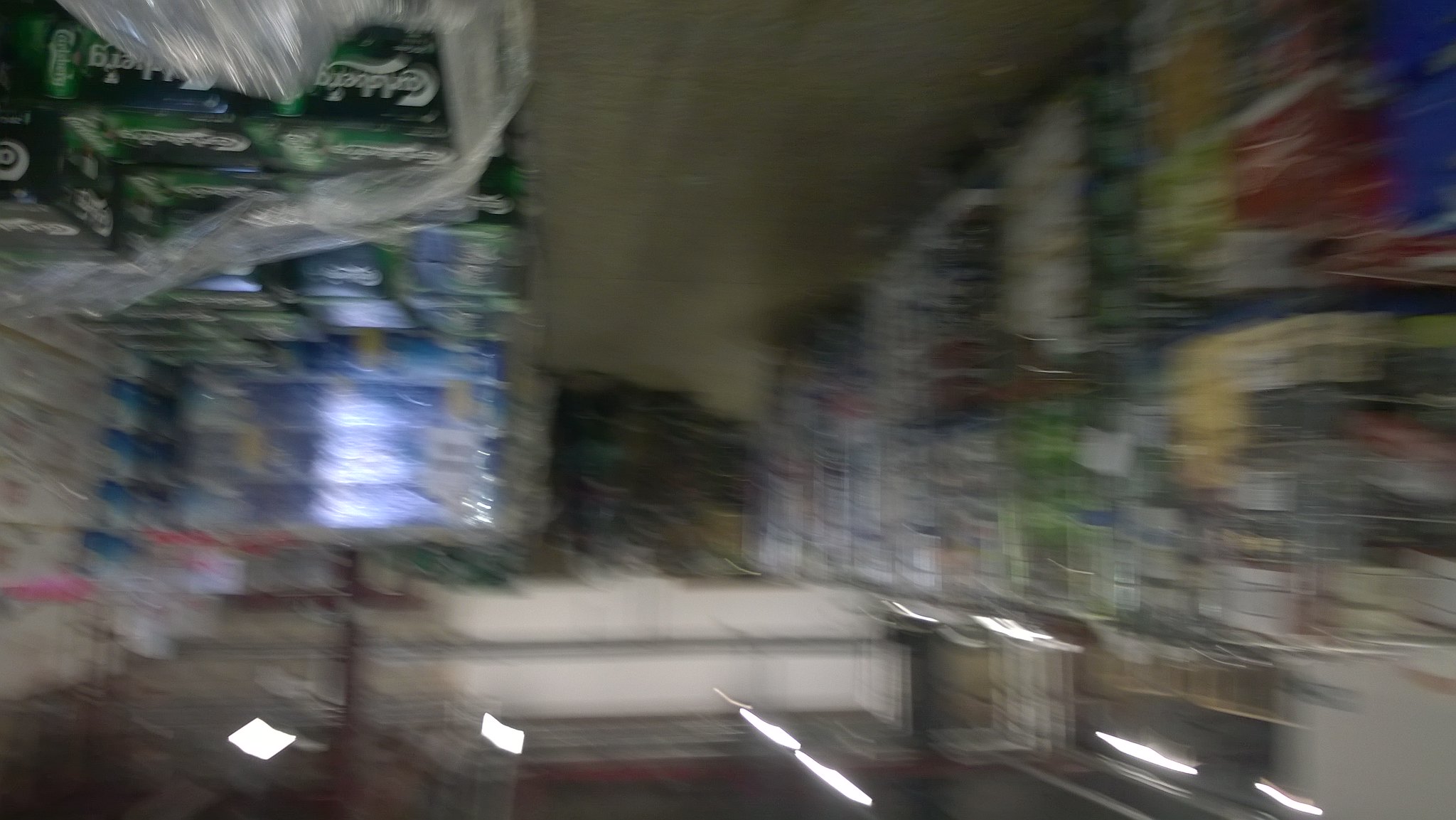This photograph is characterized by significant motion blur, making it challenging to discern specific details. The image appears to be taken accidentally while the camera was in motion, leading to a shakiness that blurs the scene. Additionally, the photograph is oriented upside down, with the floor depicted at the top and the lights and ceiling rafters at the bottom. From what can be deciphered, the scene features wrapped pallets of various products, likely taken in a store or warehouse setting. One of the more discernible elements is a shrink-wrapped pallet of green boxed drinks, possibly a 12-pack or 24-pack, though the exact product remains unclear. The left and right sides of the image are filled with a blur of colors, including blues, reds, yellows, greens, and whites, representing an array of food and drink items stacked on pallets.